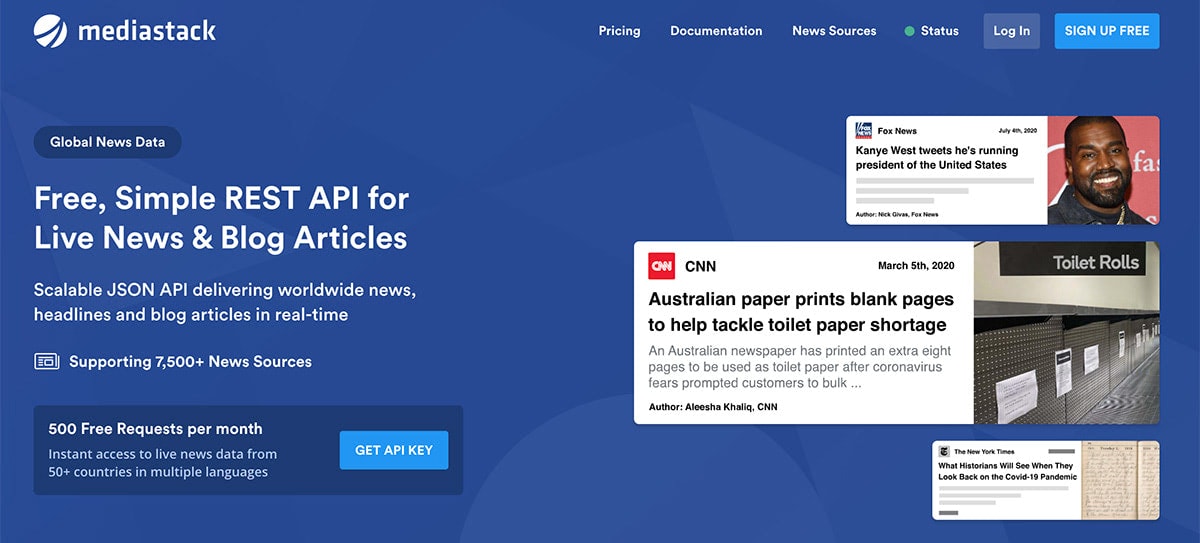**Detailed Caption for MediaStack Image:**

The background of the image is a rich, royal blue that provides a striking contrast to the white and colored elements overlaying it. In the upper left-hand corner, the MediaStack logo is prominently displayed, followed by the word "MediaStack" in clear, bold white text. To the right of the logo, there are navigational options listed in white: "Pricing," "Documentation," and "News Sources." Adjacent to these options, a green dot accompanied by the word "Status" is positioned, indicating operational status. To the right, a light gray dot marked with "Login" is visible, followed by a blue rectangle with the text "SIGN UP FREE" in all caps.

On the left side of the image, an oblong-shaped navy block showcases "Global News Data." Below this, in large, bold white type, the text reads "FREE, SIMPLE, REST API" in all caps, meant for providing access to live news and blog articles. Following this, additional information is detailed in capitalized text: "SCALABLE, JSON, API delivering worldwide news, headlines, and blog articles in real time."

Further below, multiple screen icons represent the extensive support for over 7,500 news sources. Another navy rectangle displays "500 FREE REQUESTS PER MONTH," emphasizing the generous free tier. It also mentions "Instant access to live news data from 50+ countries in multiple languages." Lastly, to the left of this information, within another navy blue block, a blue rectangle urges users to "GET API KEY."

Overall, the image effectively combines essential information and navigational prompts with a visually appealing design that underscores MediaStack's service offerings.